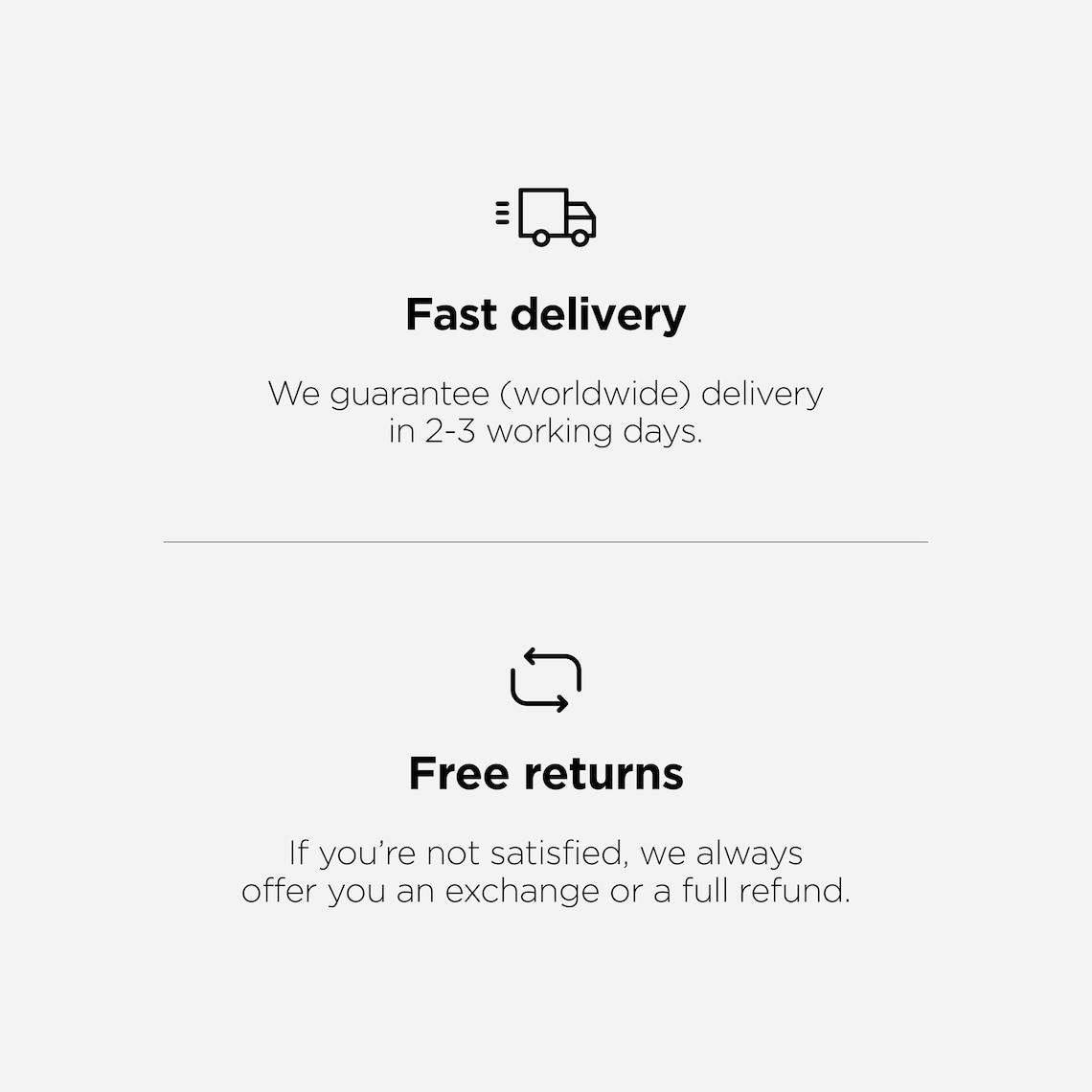The image is a screen grab resembling a promotional banner that could be from Amazon or a similar e-commerce site. The background is a light gray, providing a clean and simple aesthetic. 

At the top center of the screen, there is a small graphic of a box truck with three horizontal lines trailing behind it, symbolizing speed. Bold, black text adjacent to this graphic reads "Fast Delivery." Directly below this, it states, "We guarantee worldwide delivery in 2-3 working days." 

A line separates this section from the content below. Centered beneath is a graphic of two arrows forming a circle, representing returns. In bold text next to this icon, it says "Free Returns." Underneath, in a regular font, it explains, "If you're not satisfied, we always offer you an exchange or a full refund."

The image is devoid of any clickable buttons, hyperlinks, or additional text, emphasizing only the graphics and key messages of fast delivery and free returns. The style and layout suggest it could be from Amazon or a similar online retail platform, particularly due to the fast delivery icon that resembles those commonly found on such sites.